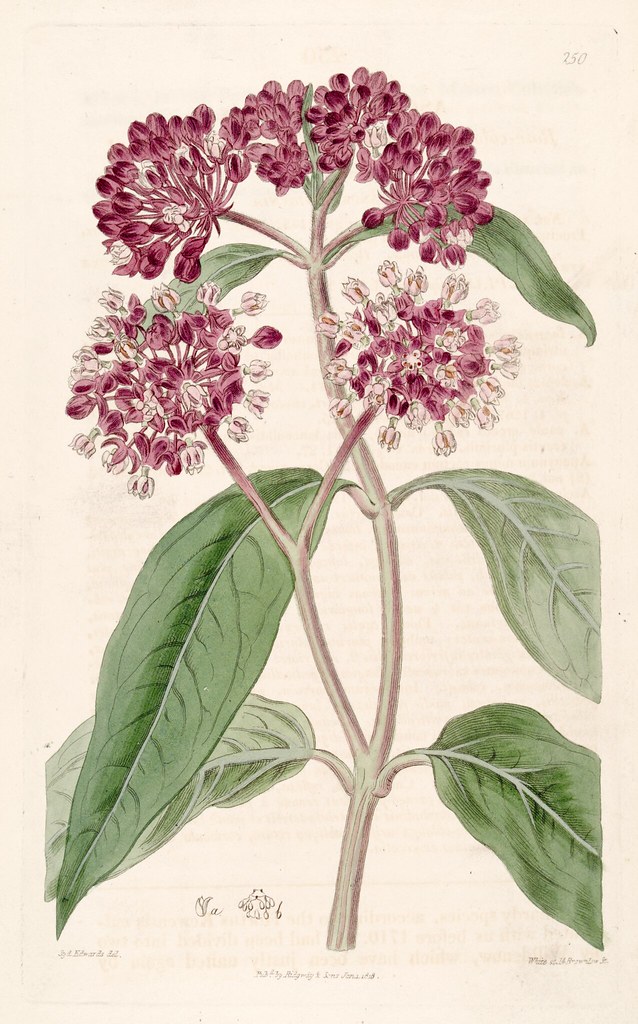This image depicts an intricate botanical drawing on tanned parchment-like paper, showcasing a flowering branch. The main feature is a cluster of maroon and light pink flowers, with six distinct clusters giving the appearance of large, round blossoms composed of numerous tiny flowers. The plant, which takes up the entire page, includes a stem adorned with six long, oval-shaped leaves that are pointed at the ends. At the top right corner of the image, the small numeral "250" is clearly visible. The bottom of the page features several cursive inscriptions and signatures, though mostly indecipherable, with hints of the name "Ridgway and Sons" and possibly the word "white." Additional faint lettering from the reverse side of the page is also visible. There are unfinished sketches of petals at the base of the drawing, contrasting with the detailed illustration of the flowering plant above, indicating the drawing's vintage and hand-drawn nature.